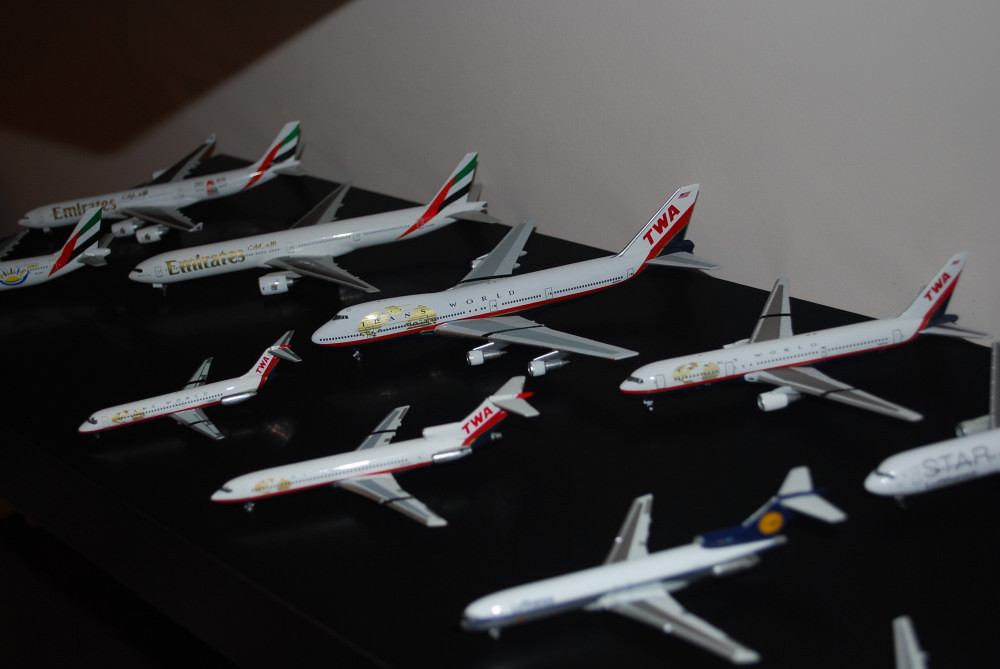This photograph features a collection of detailed miniature model airplanes arranged on a shiny black table against a plain white wall. The scene is divided into two rows, with the larger models positioned at the back and smaller ones upfront. From left to right, the models are meticulously crafted replicas of commercial jet airliners, prominently featuring two large Emirates jets on the left, easily identifiable by their white bodies with gold text and red, green, and black trim. Next to them are two large and two small TWA (Trans World Airlines) models, which sport a white body with a golden embellishment at the front, a red stripe along the bottom, and distinctive red and black detailing on the tail.

In the front row, there's a trio of smaller aircraft: two TWA models and a third with a blue tail tipped with a yellow circle, identifiable as a "Star" jet based on the barely discernible text on its side. Additionally, there is a partially visible nose of another plane in the top-right corner and the tail of another model peeking in from the bottom-left.

Altogether, this impressive display includes seven complete planes, showcasing the intricate beauty and variety of commercial aviation through these scaled-down models.